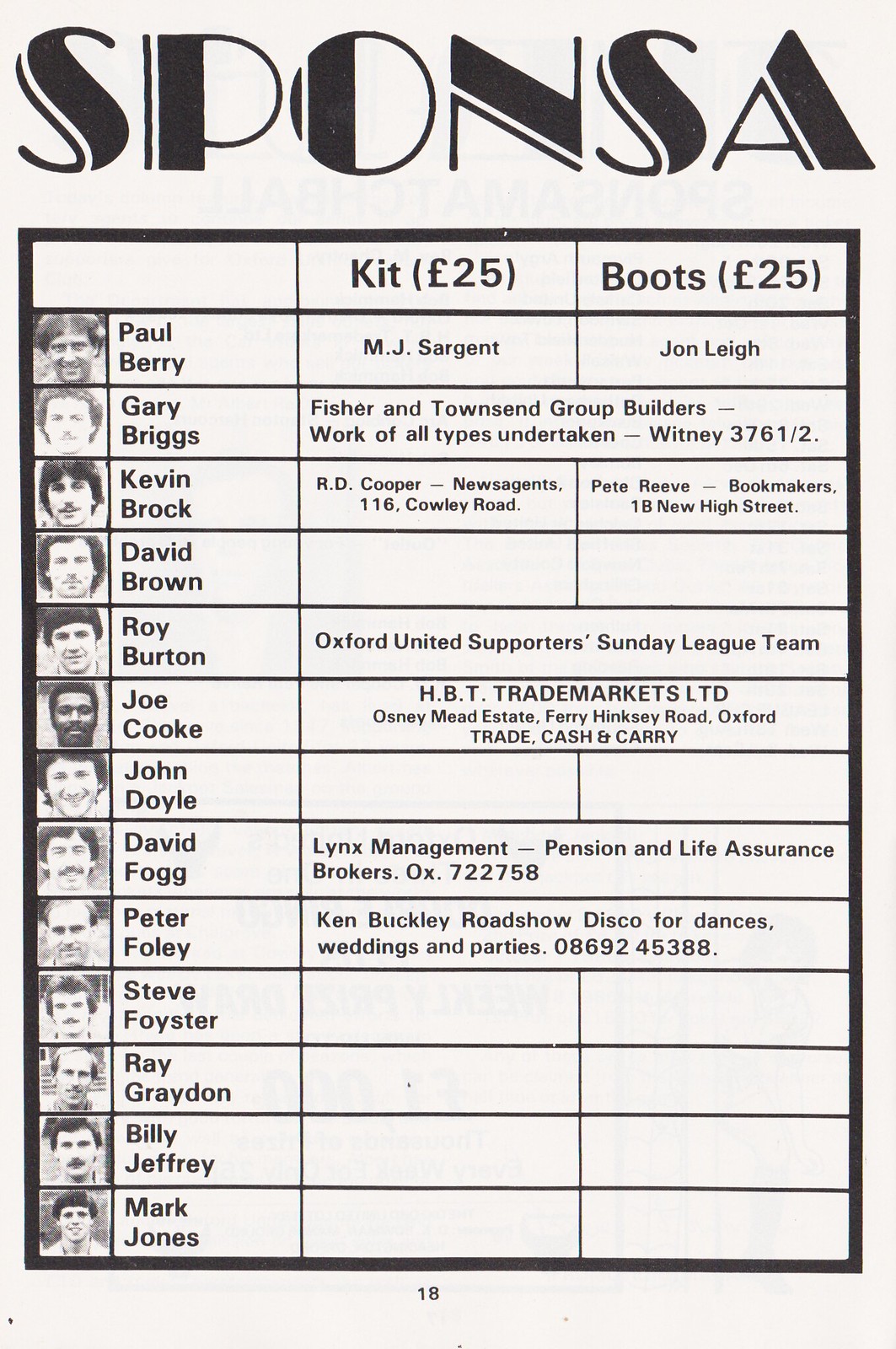The image depicts a rectangular page from a small booklet, likely around three by four inches in size, featuring sponsorship details for various individuals. At the top of the page, the word "Sponsa" is displayed prominently in old-fashioned black print against a white background. Below this title, the content is organized into three columns. The first column lists names of approximately a dozen individuals, each accompanied by a small black-and-white photograph. The second column, headed "Kit, 25 pounds," provides details of their associations or sponsors related to sports kit expenses. The third column, titled "Boots, 25 pounds," similarly lists sponsors or professional details concerning footwear costs.

The individuals listed include Paul Berry, Gary Briggs, Kevin Brock, David Brown, Roy Burton, Joe Cook, John Doyle, David Fogg, Peter Foley, Steve Foyster, Ray Graydon, Billy Jeffrey, and Mark Jones. Each row provides specific sponsorship or occupational information for these individuals. For instance, under "Kit," Paul Berry is associated with M.J. Sargent, while "Boots" lists John Lee. Gary Briggs has his details spanning both "Kit" and "Boots" columns, noting Fisher and Townsend Group Builders with additional contact information. David Fogg’s entry includes his association with Lynx Management Pension and Life Insurance, and Peter Foley is linked to Ken Buckley Roadshow, servicing discos for dances, weddings, and parties.

The page number, labeled 18, indicates its position within the booklet, adding to the impression that the booklet might serve as a specialized program or report documenting the community and sponsorship affiliations of the individuals depicted.